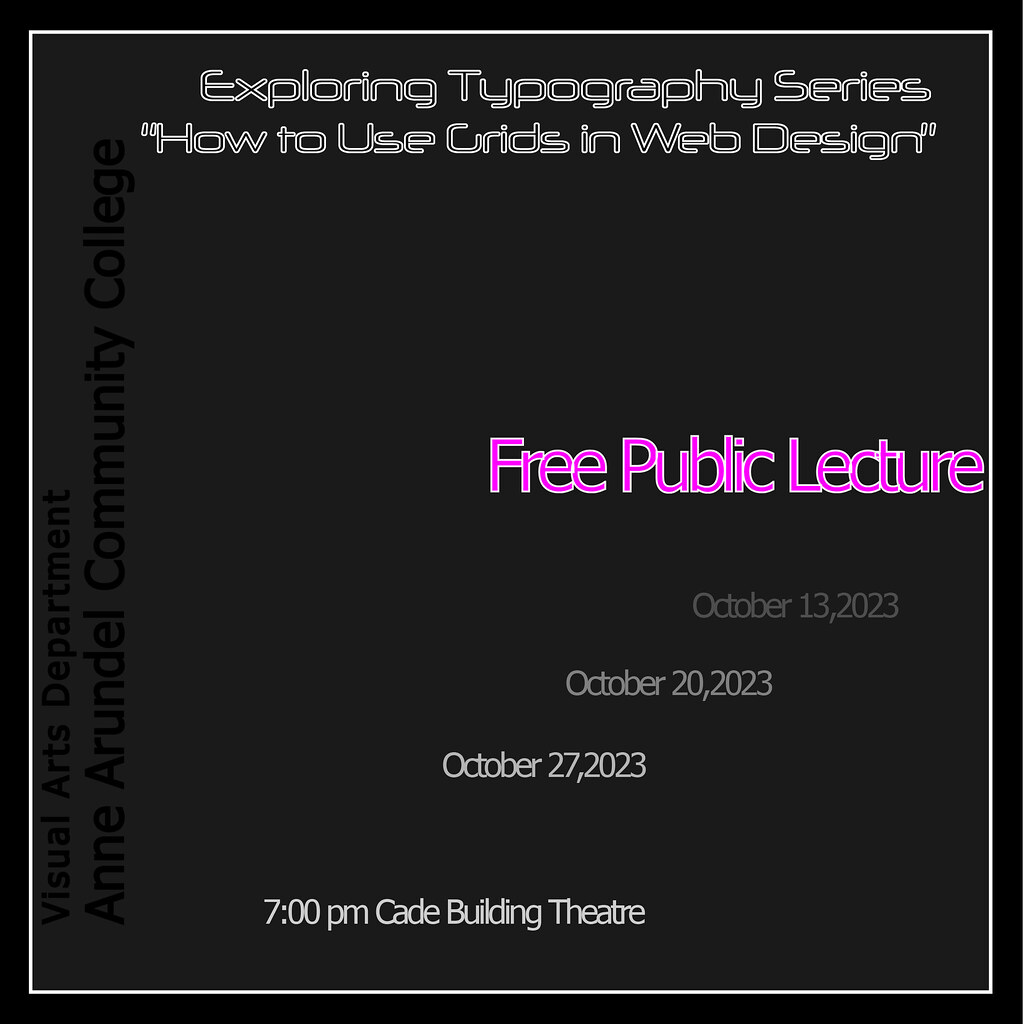The image is a detailed advertisement for a public lecture series. The background is primarily black with a white border enclosed by an additional black border. At the top of the image, it reads "Exploring Typography Series: How to Use Grids in Web Design" in white text, with "How to Use Grids in Web Design" in quotation marks. Centrally positioned in pink text with a white border, it announces "Free Public Lecture." Below this, the dates "October 13, 2023," "October 20, 2023," and "October 27, 2023" are listed sequentially from right to left as the text gets lighter in color. At the bottom, it mentions "7 PM Cade Building Theater" in white text. On the left side of the image, running vertically, it states "Visual Arts Department" and "Anne Arundel Community College," with "Anne Arundel" in a slightly larger font. The background inside the borders is a brownish-gray, adding a subtle contrast to the text elements.